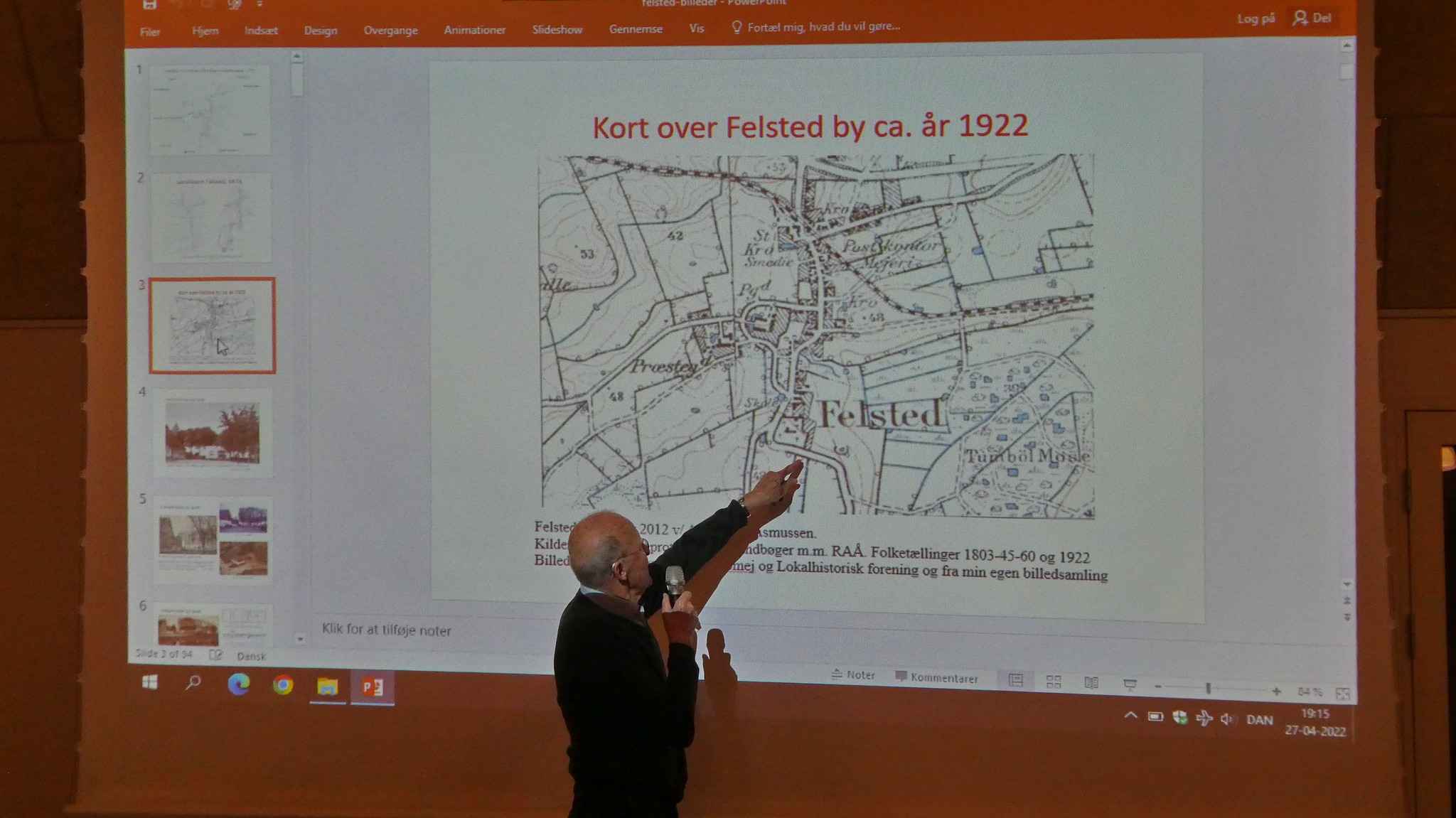An elderly white male, likely around 60 years old and bald, is seen on stage delivering a speech or teaching a lesson. He is wearing eyeglasses and a black sweater, holding a microphone in his right hand while pointing with his left to a large, projected black and white map. The map, part of a PowerPoint presentation, is titled "Court over Felstead by C.A.A.R. 1922." Beneath the map, which depicts the city of Felsted, there is some black text written in a foreign language. The PowerPoint interface is visible, indicating that the presentation was captured on April 27, 2022, at 7:15 PM. Additional slides are visible to the left side of the map, and it appears this is the third slide of a larger set, which may contain a total of either 34 or 54 slides.